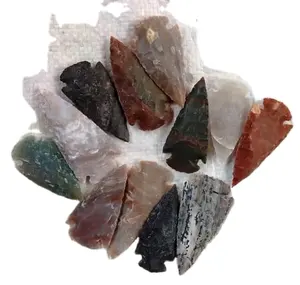The photograph depicts a collection of intricately crafted Native American arrowheads, laid out on a crinkled white surface that resembles cloth or paper. There are ten arrowheads in the foreground, arranged in varying orientations. Starting from the bottom right, there is a triangle-shaped white arrowhead with black speckles, adjacent to a dark gray or black triangular arrowhead with a small handle. Next, there is an orangish-beige arrowhead wrapped in plastic, placed with its pointed end facing down, and a red triangular arrowhead with a handle, oriented upwards. Moving left, there is a green arrowhead positioned horizontally, and next to it, a completely obscured arrowhead also wrapped in plastic. 

At the top of the arrangement, five more arrowheads lie scattered in different directions, varying in color from black to dark brown, and ranging to lighter shades such as light brown and beige. A notable dark brown or orange arrowhead is present among these. The colors of these stone artifacts include shades of black, green, red, white with black markings, dark brown, and an orangish-beige hue. This diverse palette suggests that different minerals and material types were used in their creation. Some appear to be made of obsidian, while others resemble peach crystal or other various stones. The overall display showcases the range of earthy tones and craftsmanship of these ancient tools against a textured white background.